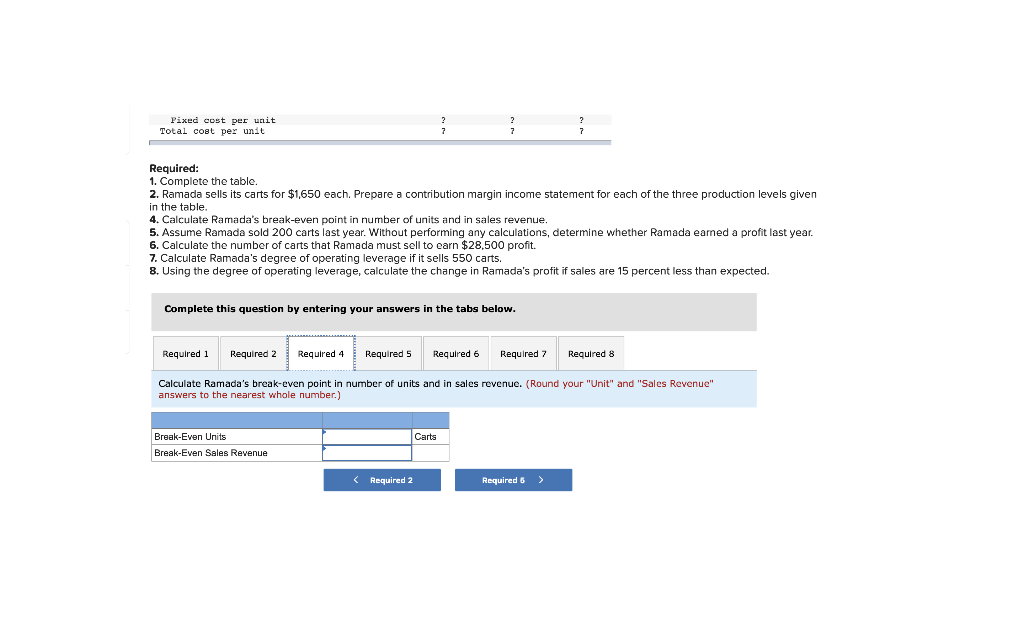The image displays a detailed analysis document pertaining to WMATA's financial performance. At the top of the document, there are headings labeled "Fixed Cost Per Unit" and "Total Cost Per Unit." Below these headings, the word "Required" is prominently displayed in bold font, followed by a list of tasks presented as bullet points. These tasks include:

1. Complete the table.
2. WMATA sells its carts for $1,650 each. Prepare a contribution margin income statement for each of the three production levels given in the table.
3. (This point appears to be missing.)
4. Calculate WMATA's break-even point in terms of the number of units and sales revenue.
5. Assume WMATA sold 200 carts last year. Without performing any calculations, determine whether WMATA earned a profit last year.
6. Calculate the number of carts that WMATA must sell to earn a profit of $28,500.
7. Calculate WMATA's degree of operating leverage if it sells 550 carts.
8. Using the degree of operating leverage, calculate the change in WMATA's profit if sales are 15% less than expected.

Following this list, another section instructs to complete the questions by entering the answers in the provided table below. Below these instructions, there are tabs labeled "Required 1, 2, 4, 5, 6, 7, and 8" to navigate through different requirements.

A blue bar beneath these tabs contains the instruction: "Calculate WMATA's break-even point in terms of the number of units and sales revenue. Round your unit and sales revenue answers to the nearest whole number." Underneath this instruction, there are two input fields labeled "Break-even Units" and "Break-even Sales Revenue." Both fields are currently empty.

Finally, there are navigation buttons to switch between various required tasks, specifically between "Required 2" and "Required 6." The current tab selected is "Required 4."